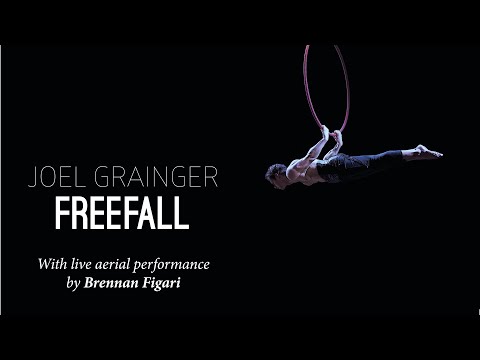The image is a dark, indoor photograph featuring a muscular, shirtless, barefoot man wearing only pants. He is an aerial performer, suspended and holding onto a large ring with his arms curved behind him, creating a striking horizontal position. The background is entirely black, making the performer and the white text stand out sharply. On the left side of the image, text in thin, almost gray white font reads "Joel Granger Freefall,” with "Freefall" entirely capitalized. Below this, in italicized white font, it reads, "With live aerial performance by Brennan Figabi." The performer's form and the text are the sole visible elements, emphasizing the striking contrast and highlighting the intensity and grace of the aerial performance.